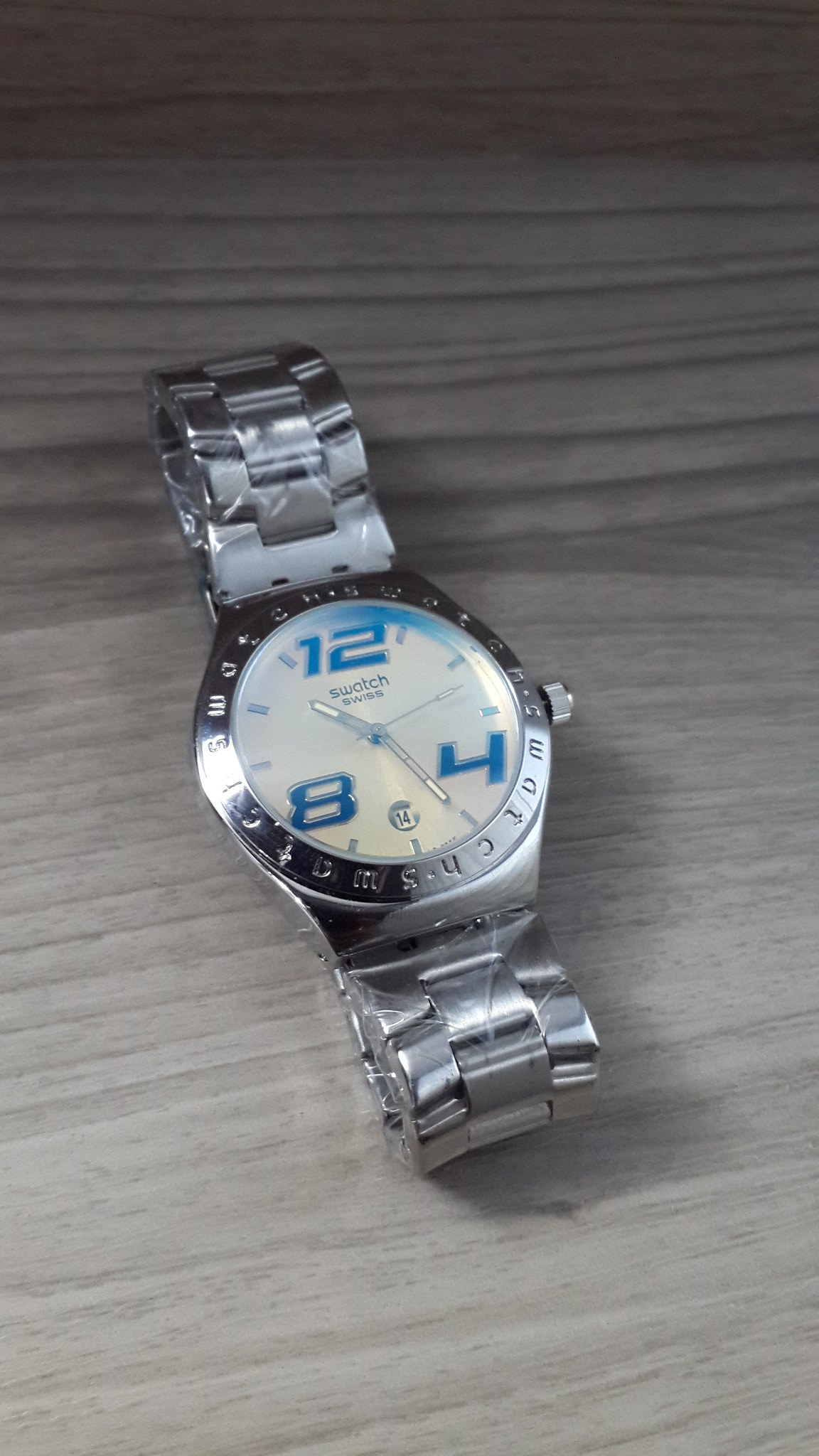This color photograph, presented in a long thin portrait orientation, features a Swatch Swiss wristwatch elegantly placed on a grey wooden grain textured table or desk. The watch has a silver stainless steel link band, partially covered in a plastic cellophane-style material, which appears crinkled in some areas. Its white or light grey face prominently displays large blue numerals at the 12, 4, and 8 positions, with the bold, italicized 12 underlined by the Swatch logo and "Swiss" inscription. The hour, minute, and second hands are silver with a phosphorescent glow-in-the-dark edge. The hands are currently indicating approximately 10:25, and the second hand is positioned near the 10. At the 6 o'clock position, a small window shows the date counter with the number 14 visible inside. The outer edge of the watch face is adorned with the "Swatch" branding, and a winding knob is situated on the right side of the dial, adding a functional and aesthetic touch to this sophisticated timepiece.